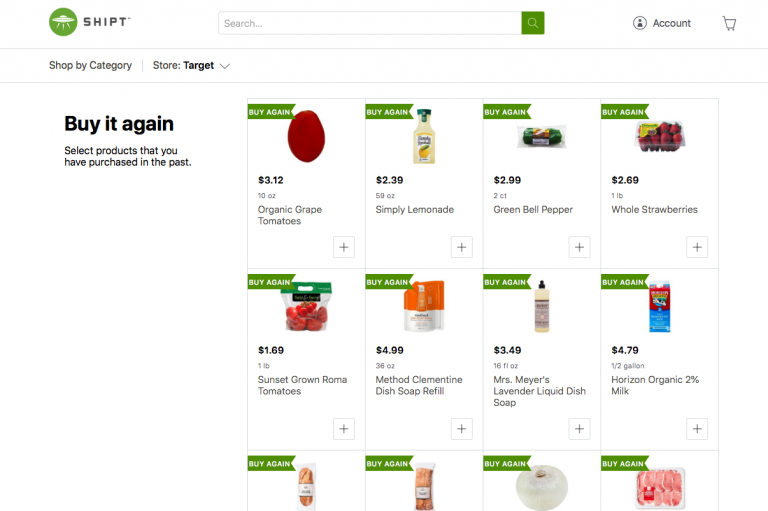This cropped screenshot of the Shipt website's desktop version primarily displays the site's user interface during the shopping process. In the top-left corner, the Shipt logo is prominently featured. Centrally located near the top of the page is a search bar, with the placeholder text "search" in small gray letters and a green box with a white magnifying glass icon on its right side. 

Towards the top-right corner, an account icon accompanied by the word "Account" in bold gray letters is visible, followed by a shopping cart icon further to the right. Below the primary navigation area, the page features a "Shop by category" label on the left, and directly to its right, the word "Target" is displayed in bold black font within a dropdown box that allows users to switch stores.

The main content area of the webpage has a clean, white background. On the left side towards the top, a "Buy it again" section is highlighted in bold black letters, inviting users to "select products that you have purchased in the past." The section showcases a vertical list of products, arranged in rows of four items each. Each product entry includes a "buy again" banner in green at the top-left corner of the product image, followed by the item's price, weight, and description.

The first product listed is organic grape tomatoes, marked by an image of grape tomatoes and the green "buy again" banner. Similarly, the second product is Simply Lemonade, showcased with a small photo, price, weight, and name. This layout is consistent across the 12 products visible in the screenshot, providing a straightforward and organized shopping experience.